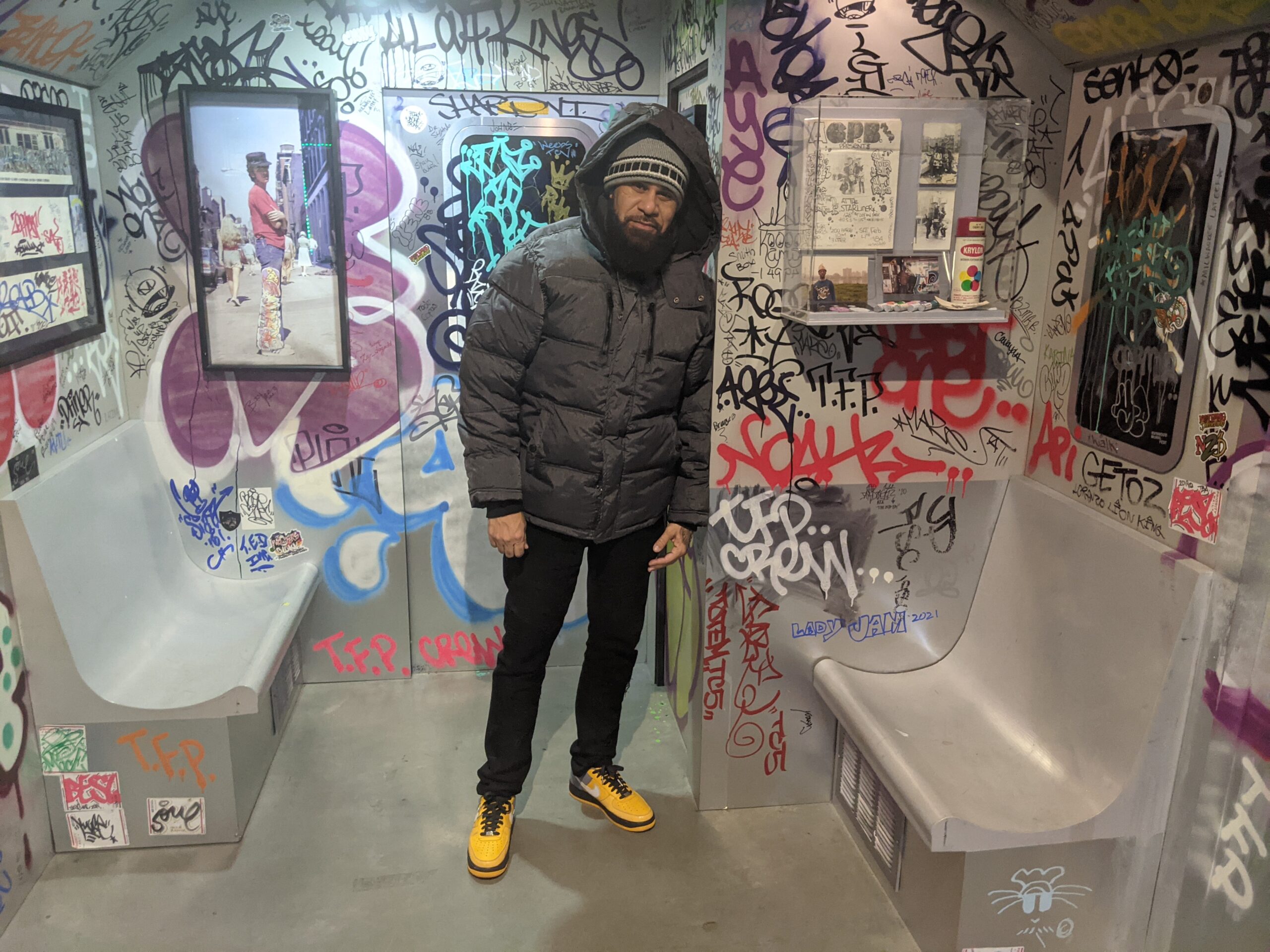The photograph depicts a man standing in the middle of what appears to be a meticulously recreated subway car interior, likely a museum display given the context. The scene is detailed with two gray, metal benches on either side of the man, each carved out in a booth-style format. The entire backdrop is alive with a vibrant array of graffiti in myriad colors—whites, greens, pinks, reds, and teals—covering every inch of the walls and doorway.

The man, positioned centrally by a doorway, is adorned in a puffy, dark gray jacket with a hood over his head, beneath which he wears a gray beanie, complementing his black pants. His bright yellow shoes starkly contrast the grayscale environment around him. His facial features are defined by a mustache and thin beard, with his expression resting between a neutral stance and a slight smirk. One key detail supporting the museum display theory is the presence of a lucite-encased display shelf to the right of his head, containing a spray paint can and other artifacts. Additionally, to his left, there is a framed picture of another man standing on a street, further enriching the scene.

This scene's overwhelming display of graffiti—mostly tags and names—contributes to a strong urban aesthetic, making the interplay between the man's modern attire and the graffiti-strewn environment a point of fascination for viewers.